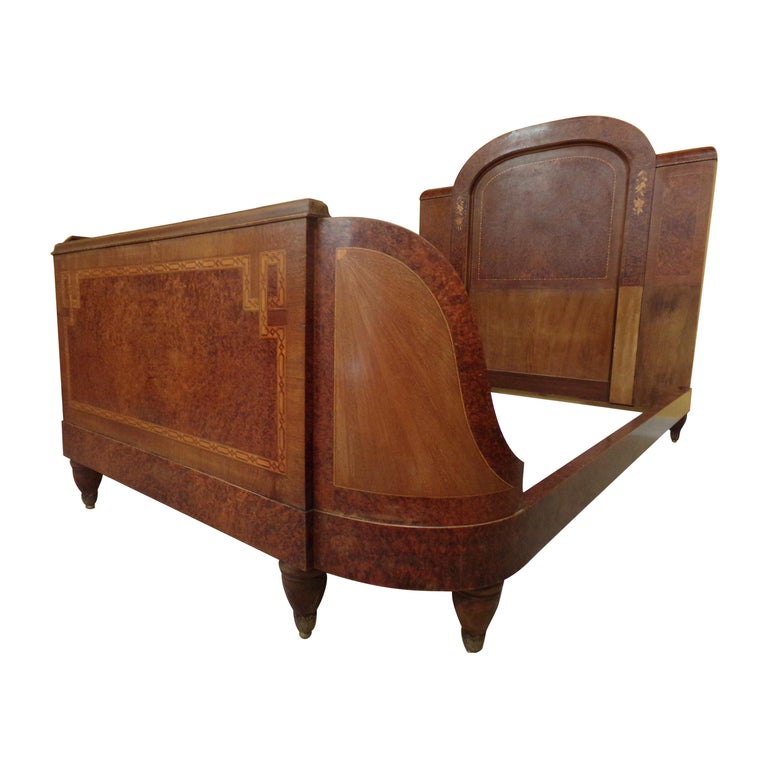The photograph depicts a wooden bed frame set against a completely white background. The frame, devoid of any mattress or box springs, is presented from the foot of the bed looking towards the headboard and slightly angled toward the side. Made from wood, possibly mahogany, the bed frame exhibits a rich brown coloration with hints of reddish and lighter brown tones throughout its structure. The prominent headboard and substantial base of the frame feature subtle designs—a light brown stencil forming square-like patterns. The frame stands on visible legs—two at the foot and two at the headboard, with just a glimpse of the fifth supporting leg on the other side, indicating a standard yet ornate design. The image, centrally composed with no text or additional elements, appears to be taken to showcase the craftsmanship and detailed features of the antique-looking bed frame.